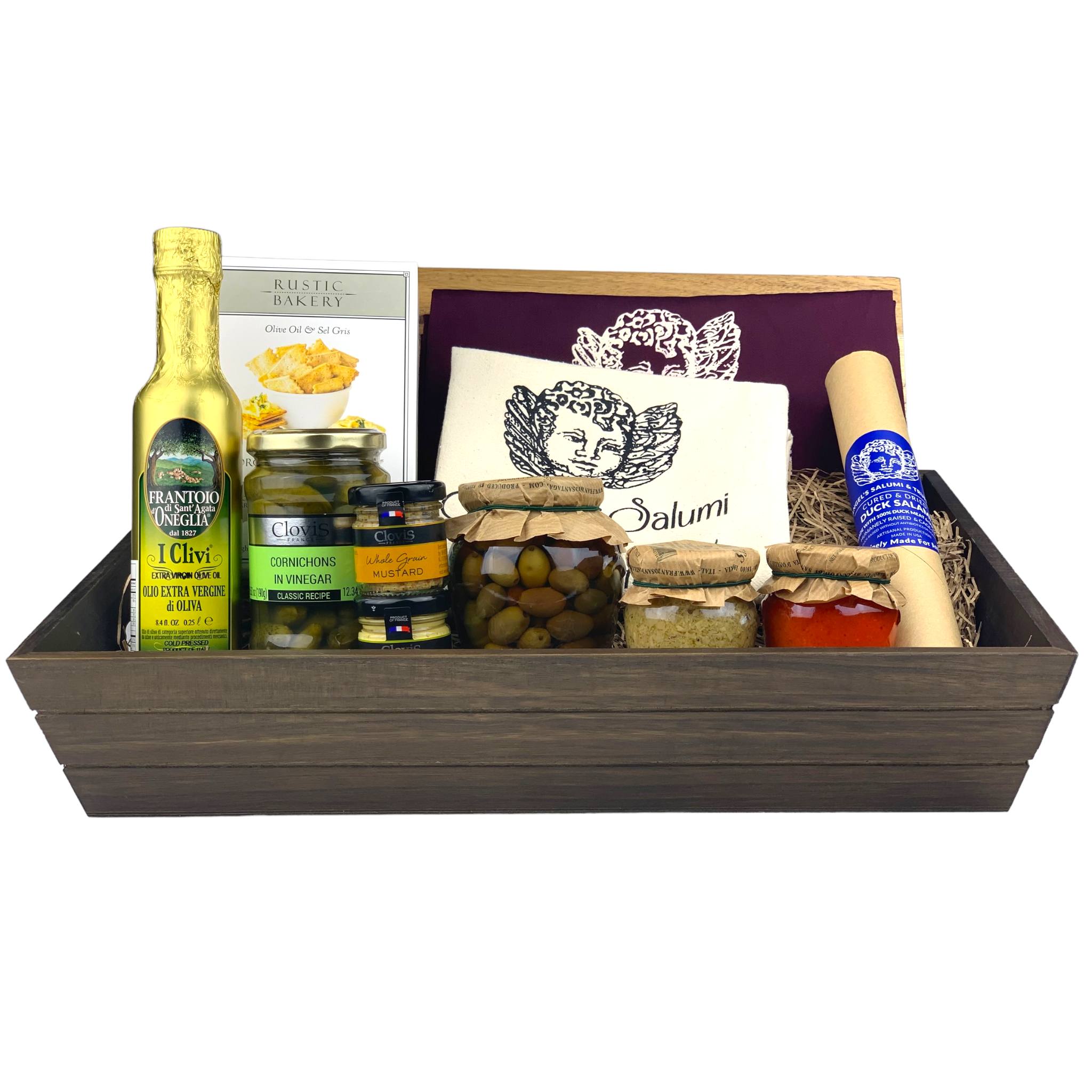The image displays a dark wooden, rectangular basket designed like an open tray with sides approximately four to five inches high, set against a completely white background. The basket has three horizontal wooden slats on its front and is filled with brown straw, on which a variety of gourmet food items are neatly arranged.

On the left side of the basket is a bottle of extra virgin olive oil labeled "Frantoio Oneglia Clivi," adorned with gold foil around its top. Behind this bottle is a book titled "Rustic Bakery," featuring a picture of a bowl with food on its cover. In front, to its immediate right, are two smaller, clear jars: one containing cornichons in vinegar and the other holding whole grain mustard.

Situated in the middle of the basket is a larger jar filled with green olives, alongside another smaller jar containing a light, flaky substance, possibly rice. Further to the right is another small jar with a red substance, potentially pimentos. The most prominent item to the far right is a package with a blue label that reads "duck salami,” featuring a cherub illustration on a small card attached to it.

This thoughtfully curated assortment of items appears to be a gourmet gift hamper, elegantly presented and filled with culinary delights.